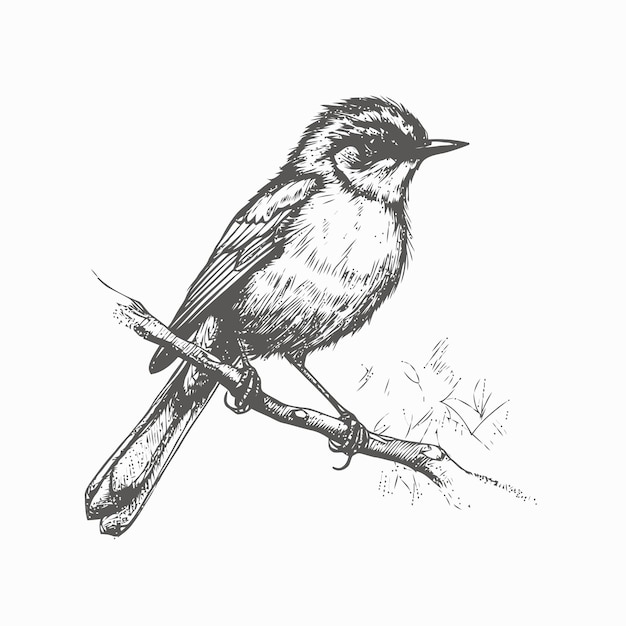This is a detailed black and white ink drawing of a sparrow, presented against an ostensibly white background, although there may be an off-white tint that is subtle and possibly imaginary. The bird, shown in profile facing to the right, features intricate details like a sharp, short beak, one visible eye, and a plumage on its head shaded in brown tones. Its small, closed wings and long tail feathers, which extend down to the lower left, are also evident. The sparrow's light-colored breast contrasts with the alternating brown and white striped feathers on its side. It perches on a thin branch that angles from the lower right to the upper left of the image, with some cross-hatching suggesting shadows and additional branches in the lower right. The drawing includes no borders or text, and no other animals are depicted.